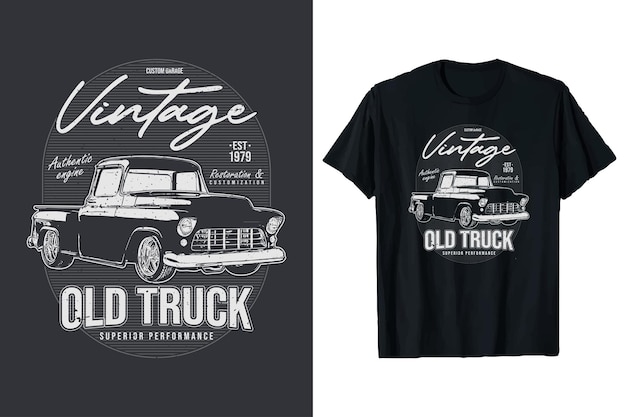The image features a black t-shirt with a ribbed collar and short sleeves on the right side. The centerpiece of the t-shirt is a circular, iron-on transfer depicting an old-style truck with a short bed and a Cadillac-like front. At the top of this design, there's small white text that reads "Vintage," followed by "EST 1979." Below that, cursive text states "Restoration and Customization," along with "Antonio's Engine," and then "Old Truck," all in capital white letters with a minor 3D effect. Underneath the truck image, the text "Superior Performance" is prominently displayed in all capital letters. On the left side of the image, there is a larger, zoomed-in version of this same decal framed in black, emphasizing the intricate details of the design and text.